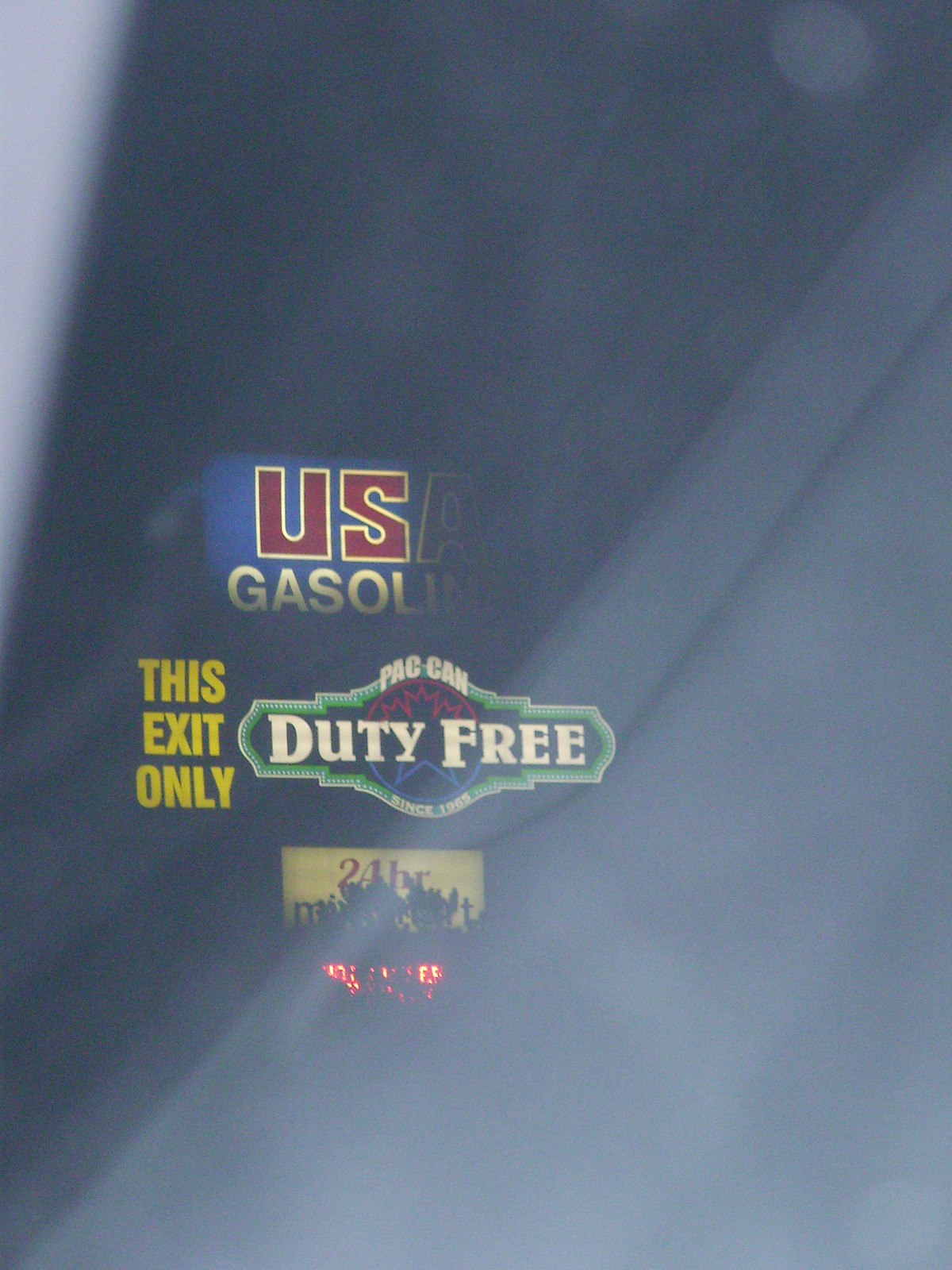This nighttime photograph, taken from a moving vehicle, captures a series of billboards flanking a highway exit. The topmost billboard stands out with bold red letters trimmed in white against a blue backdrop, spelling "USA," although the 'A' is partially shadowed. Below it, the word "gasoline" is displayed in white text; however, only "gasol" is fully illuminated while the remainder fades into shadow. Underneath this billboard, a green diamond-shaped sign with white letters reads "pack can duty free since 1965," possibly advertising a liquor store. To the left, another yellow sign proclaims "this exit only," indicating the exclusivity of the services provided at this exit. Partially obscured and somewhat degraded by dirt and possible graffiti, a final sign at the bottom suggests "24 hours," with hints of additional text that is difficult to decipher, potentially a "market" or "motel." Despite the blur and glare of lights, this vivid nighttime scene of illuminated billboards offers a glimpse into roadside advertising and navigation.